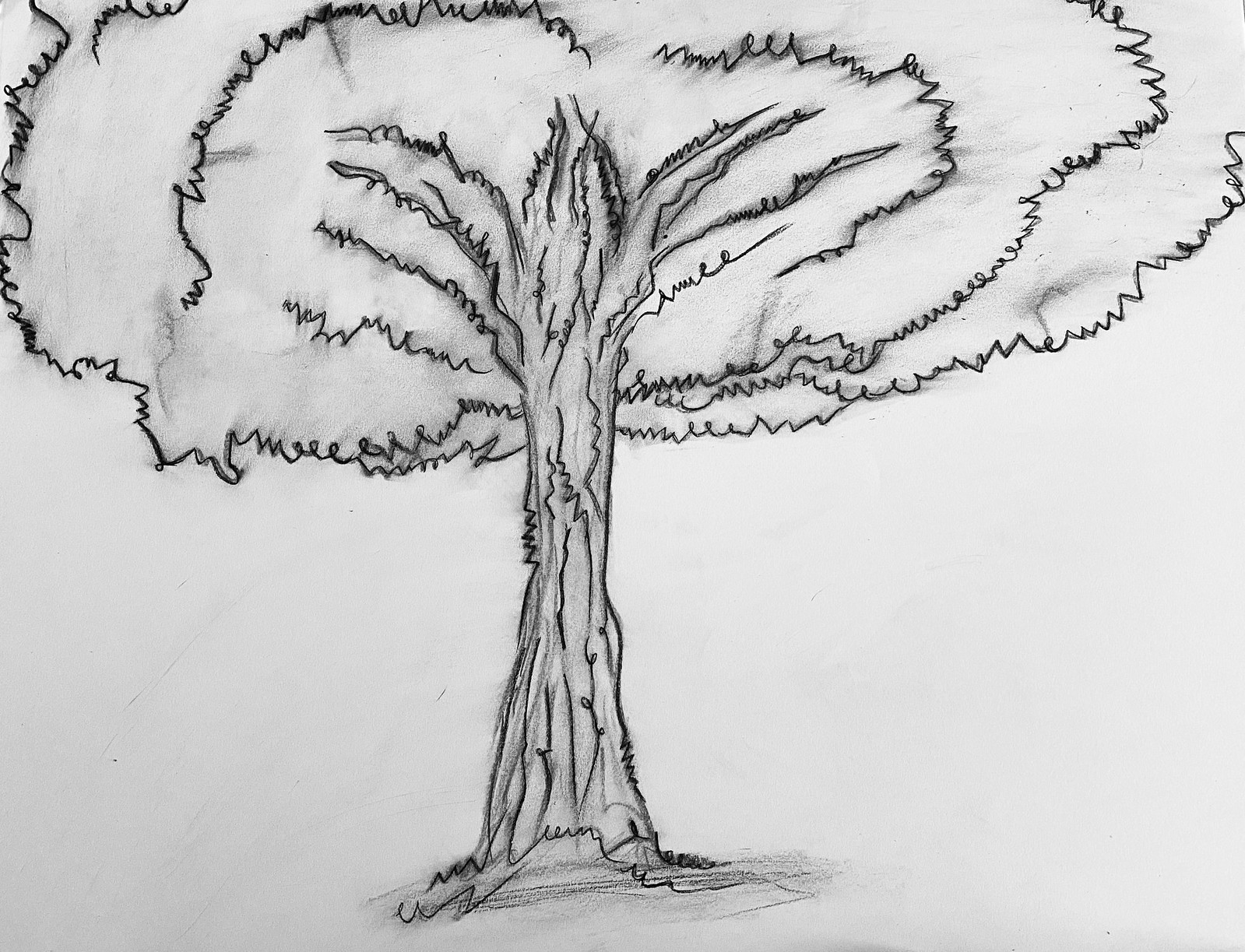This photograph showcases a meticulously detailed black pencil drawing on a crisp white sheet of paper, featuring a majestic and robust tree. The tree's thick and powerful trunk anchors the image, grounded by an intricate array of grey-shaded roots at the base. Above, the expansive canopy dominates the upper half of the drawing, with leaves outlined in delicate, squiggly lines. The artist's technique includes three distinct lines on each side of the tree, highlighting its structural segments. Various branches emerge intricately from the trunk, extending outward to support the sprawling foliage, each crafted with the same squiggly line technique, creating a sense of organic growth and symmetry.